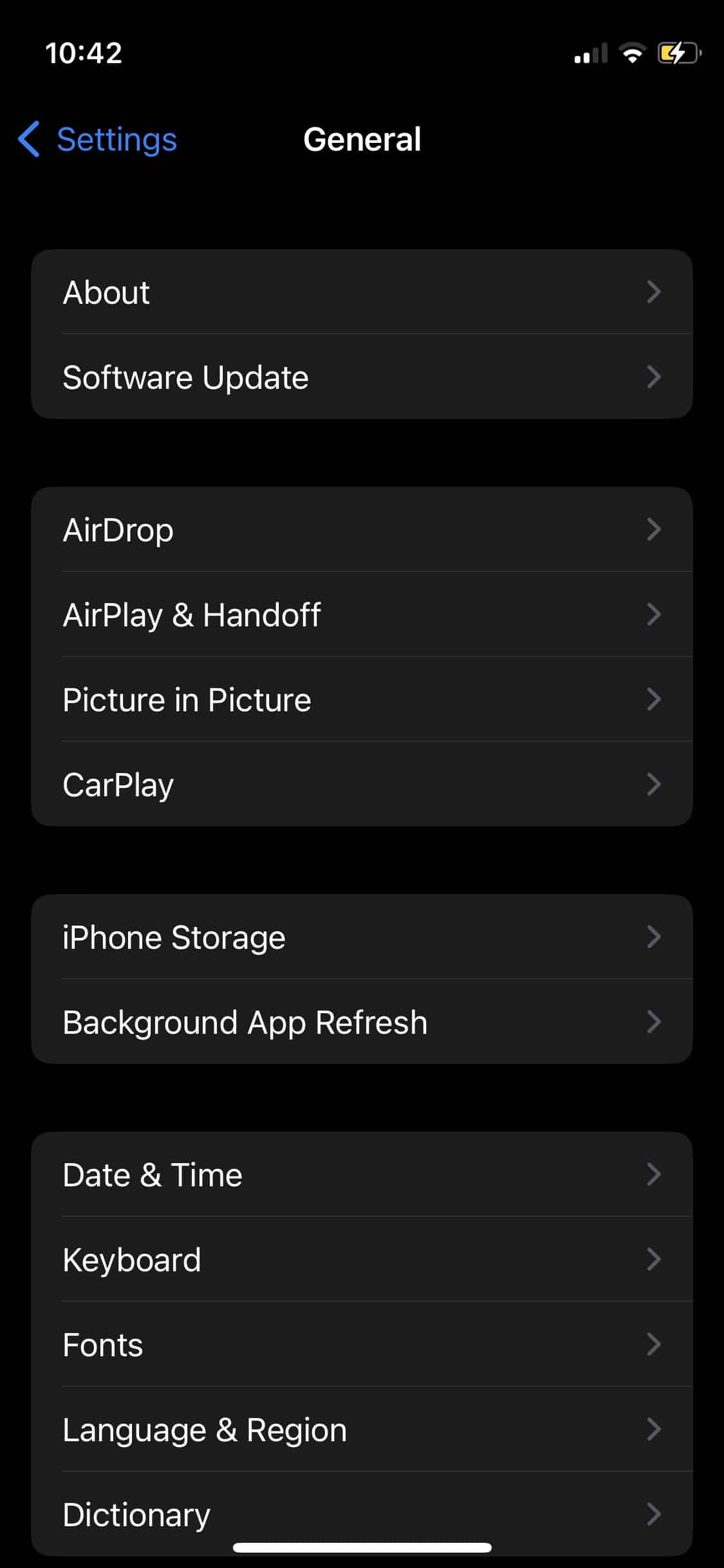The image is a vertically oriented screenshot featuring a black background. At the top left corner, the time "10:42" is displayed. On the opposite side, top right, various status icons are shown: two bars indicating the battery level, a Wi-Fi or internet connectivity symbol, and an icon with a lightning bolt, suggesting that the device is currently charging.

Just below this status bar is the header section containing navigation and section identifiers. The word "Settings" appears in blue with a capital "S" followed by lowercase letters. To the left of "Settings" is a blue back arrow icon. To the right of "Settings," the word "General" is displayed in white with a capital "G."

Beneath the header are several menu items, each aligned to the left edge of the screen:
1. "About" with a capital "A".
2. "Software Update" with capital "S" and "U".
3. After a slightly larger gap, "AirDrop" is listed, with both "A" and "D" capitalized.
4. Finally, "AirPlay & Handoff" appears, with "A", "P", and "H" capitalized.

Each menu item is presented in a clean, organized manner, enhancing clarity and ease of navigation.